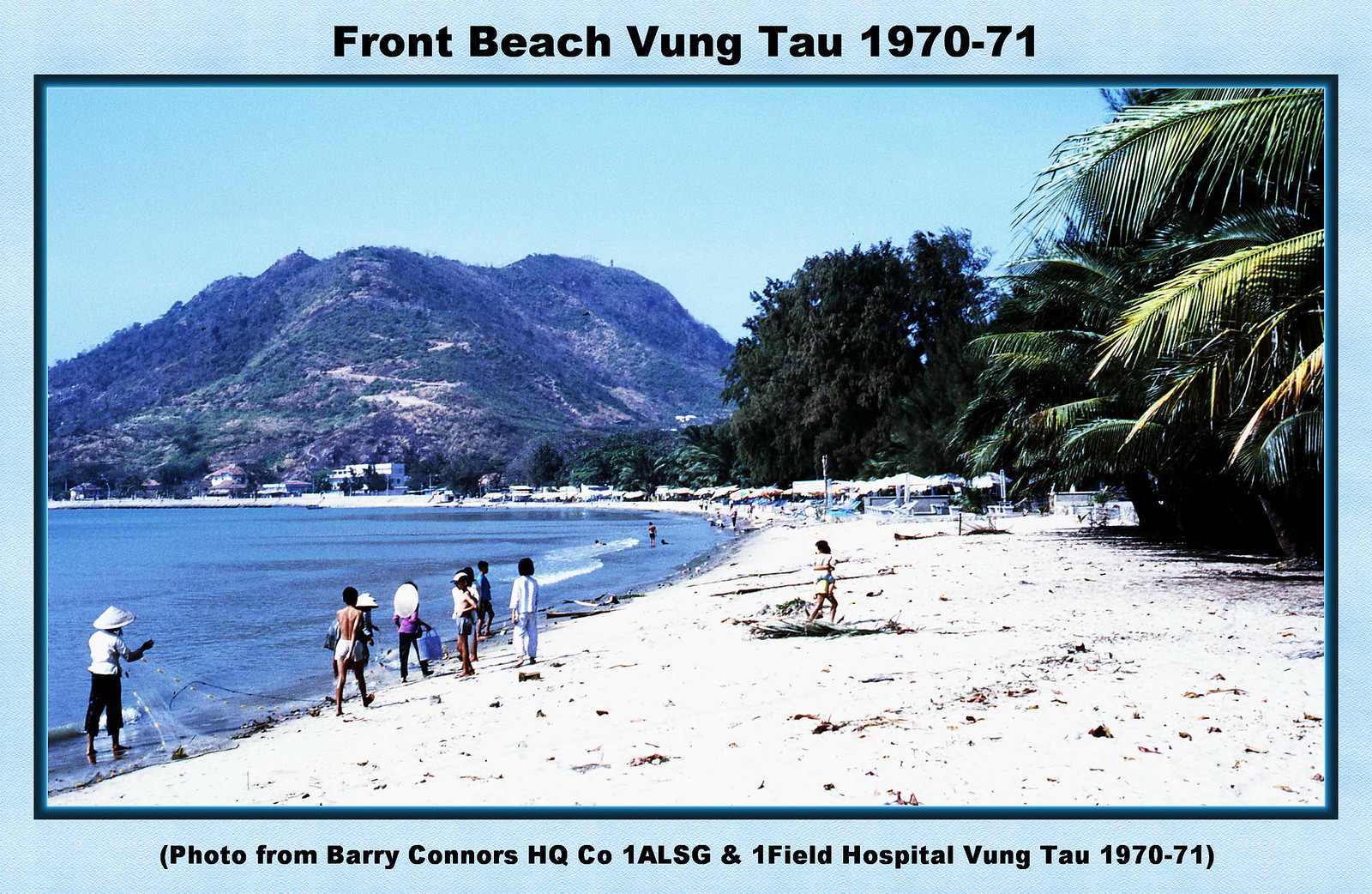The horizontally aligned rectangular picture, enclosed in a light blue border, features a nostalgic snapshot titled "Front Beach, Vung Tau, 1970-1971" at the top. The image captures a serene coastal scene with a pristine clear blue sky above. To the left, a vast expanse of ocean gently laps against a curved shoreline, where several people stand, some wading in the shallow waters while others walk or gather on the sandy beach. There are also a few visible under umbrellas situated along the curve of the beach. In the background, tall, verdant hills adorned with trees rise up, and a few houses are nestled at the foot of these hills. The right side of the picture presents several palm trees stretching out from the upper portion of the photo, framing the idyllic scene below. At the bottom of the image, in black text, is a credit notation: "Photo from Barry Connors, HQ Co., 1ALSG and Onefield Hospital, Vung Tau, 1970-71". This vintage photograph, with its detailed depiction of a tranquil beach, hints at its creation in the 1970s.